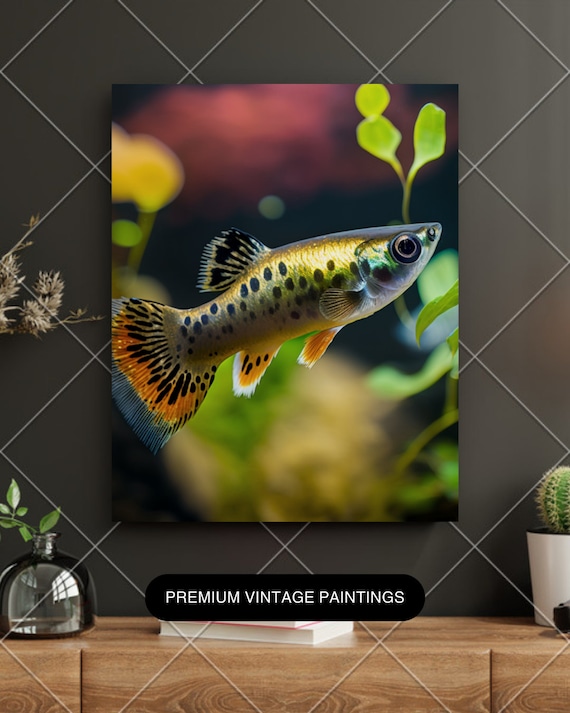The image is a digitally enhanced, full-color photograph of a painting displayed on a vertically rectangular canvas without any distinct border or background. The painting is set against a gray wall overlaid with a crisscrossing diamond pattern. Positioned at the bottom is a black banner that reads "premium vintage paintings" in white text. The scene includes a wooden countertop with decoration: a white vase holding a small cactus in the lower right corner and a silver vase with a green sprig in the lower left. Dominating the scene is a brightly colored, digitally created depiction of a tropical fish. The fish, portrayed underwater amidst green aquatic plants, has a primarily golden-yellow body with black speckles, translucent head, and black eyes. Its fins are a mix of orange and yellow, accented with black dots. The vividness and detail suggest digital manipulation, contributing to the high-gloss, high-quality appearance, reminiscent of promotional material for premium vintage artwork.